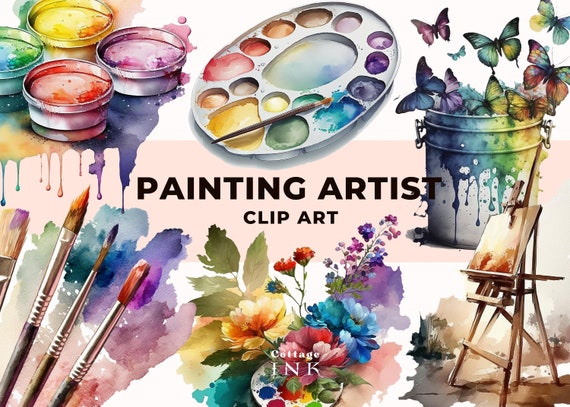The image, captioned "Painting Artist Clip Art," features a variety of vibrant and artistic elements carefully arranged on a smooth, likely printed white background. Dominating the center of the image is a paint tray filled with an array of colors ranging from purple, blue, and green to yellow, red, and orange. A paintbrush dipped in blue paint rests within the tray, adding a dynamic touch. 

In the upper left corner, there are multiple cups in yellow, purple, green, blue, and red, adding to the colorful display. Adjacent to these is a cluster of watercolors in green, blue, and purple. The bottom left corner showcases four different styles of paintbrushes, including a very thin brush in the middle, two medium-thickness brushes, and a commercial paintbrush on the far left, each accompanied by their respective paint colors.

Towards the right of the image is a noteworthy bucket, off-white in color, with bright, multi-colored butterflies (blue, violet, and green) emerging from it, some with rainbow-stained glass wings. Below the bucket is a canvas, indicating the presence of an easel. At the bottom of the image, there is a bouquet of flowers among a palette of paints, reinforcing the theme of artistry and creativity.

Overall, the composition is not only rich in detail and color but also visually engaging, capturing various aspects of art supplies and painting in a detailed and lively manner.